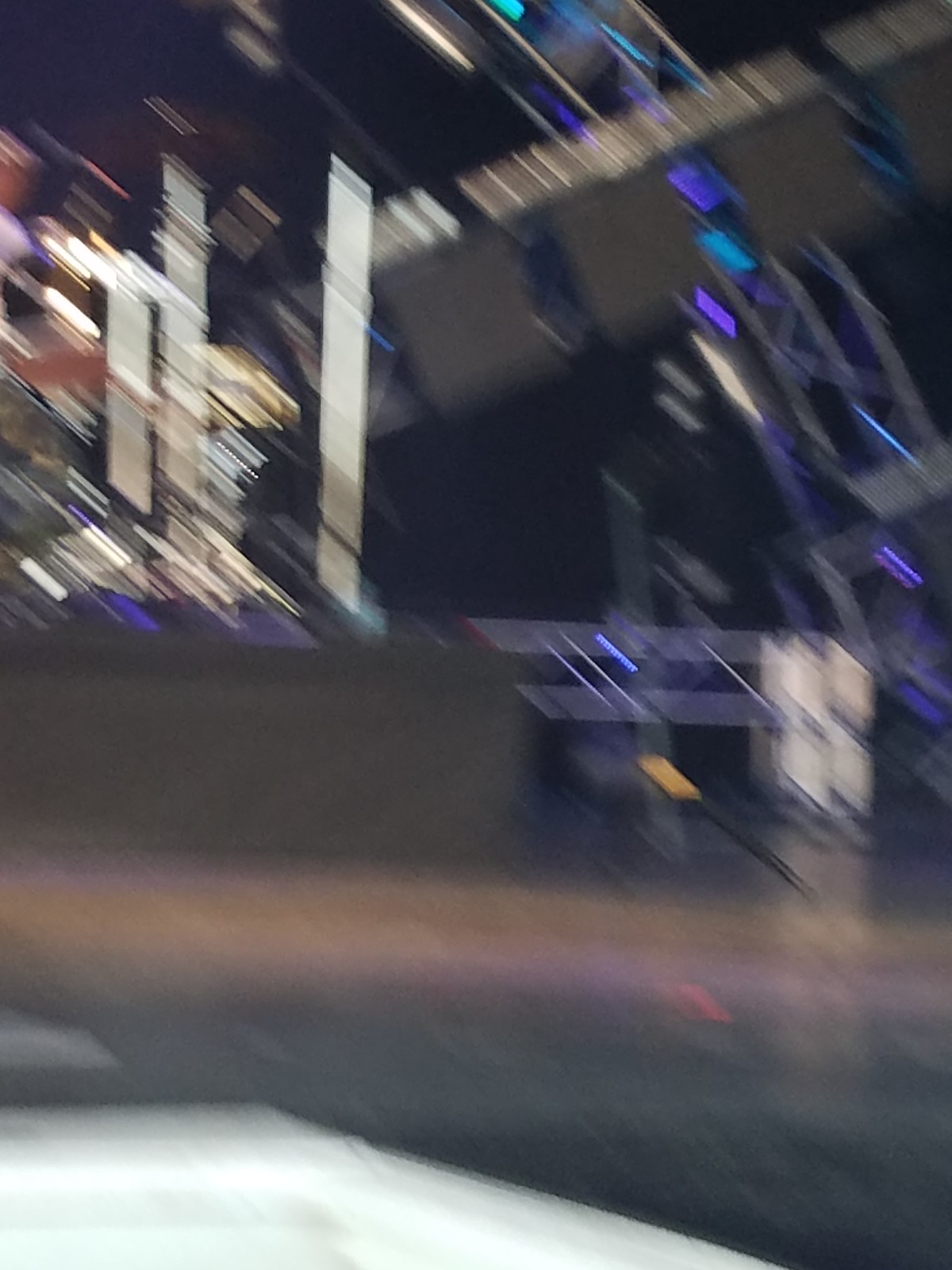This image captures an extremely blurry nighttime scene that evokes the atmosphere of a lively event, potentially at a fair or theme park. The shot appears to be taken with a moving camera, resulting in numerous streaks of light, primarily creating diagonal and vertical lines. These stripes of blue, purple, and white light add an abstract, almost chaotic feel to the image. Dominating the background is what seems to be a Ferris wheel, with its arc descending from the top center to the center-right of the frame. The Ferris wheel is enveloped in a haze of gray but is punctuated by the light trails. In the foreground, there's a vague flat white surface, possibly part of a stage or a road barrier, with a bluish fence or barrier and a significant silver metal beam that stretches from the left to the right across the top. A drummer is faintly discernible in the distant background, hinting that this could be part of a concert set. The overall scene is chaotic yet intriguing, capturing the essence of a vibrant, colorful night filled with music and movement.